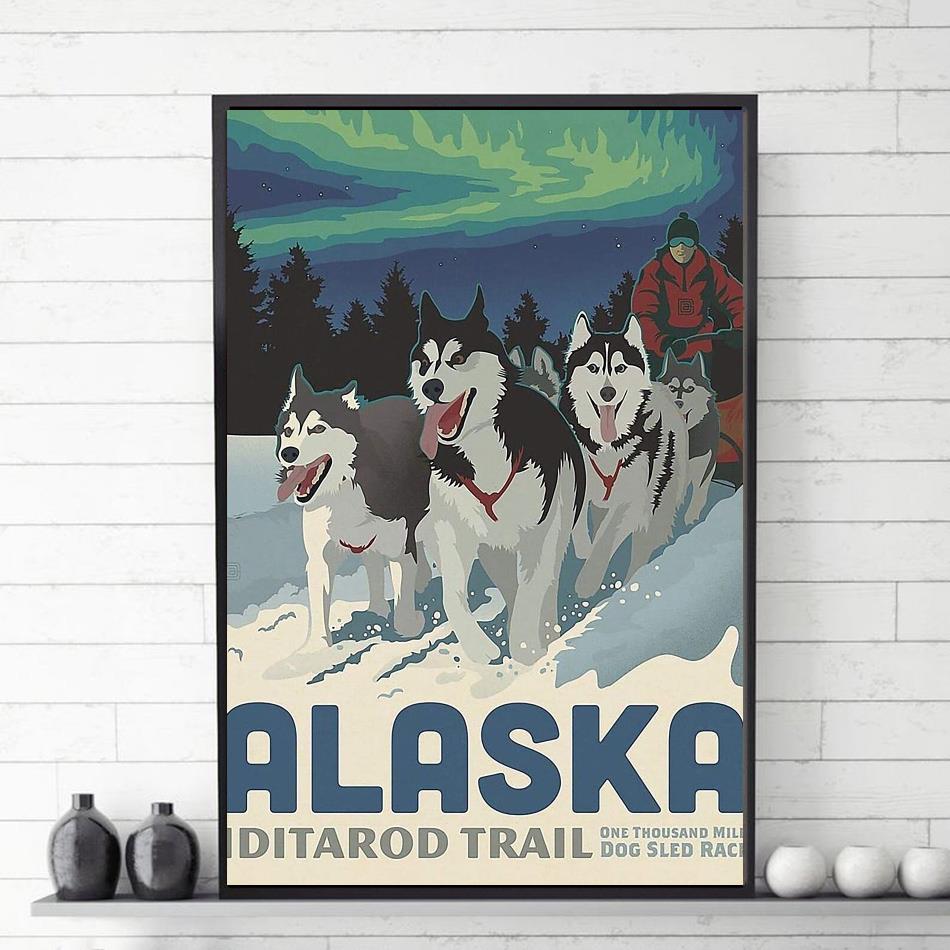The framed poster showcases the Alaska Iditarod Trail, a legendary 1,000-mile dog sled race. Positioned against a white brick or paneled wooden wall, the artwork sits on a small gray shelf flanked by two black ceramic vases and three oval-shaped white vases. The poster, outlined in black, is a cel-shaded painting that vividly captures the essence of the event. 

In the central focus, five eager huskies with their tongues out and red collars are vigorously pulling a sled. The musher, clad in a puffy red jacket, black knit cap, goggles, and ski glasses, stands gripping the sled. Underneath the illustration, the text reads "Alaska" in rounded blue letters, “Iditarod Trail” in green, and "1,000 Mile Dog Sled Race" in gray.

The background features a silhouetted evergreen forest under a dark, starry night sky illuminated by shades of the aurora borealis in blue and green hues. The snow-covered ground transitions from blue to white, adding depth to the scene. The picture as a whole exudes the style of a classic travel poster, now trendy and appealing, capturing the adventurous spirit of the Iditarod.